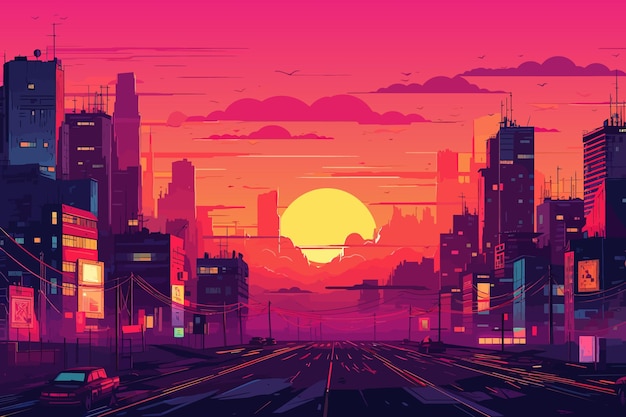The painting captures a vivid cityscape at sundown, with a highway running through the center of the scene. Dominating the composition is a bright orange sun half-obscured by the skyline. The sky showcases a gradient of colors, starting with a light pink just above the horizon, deepening to darker pink and orange hues higher up, punctuated by rolling clouds. Some of the clouds are particularly dark pink, contrasting with the lighter sky. To the far right, there's a singular cloud tinged with shades of dark purple.

Buildings flank both sides of the highway. They start off as dark silhouettes, almost black, with sporadic yellow lights indicating lit windows. As they approach the sun, they adopt a warmer palette of purple and pinkish tints, ultimately appearing light orange closest to the sun's glow. The highway itself is depicted with streaks of black and orange, interspersed with purple blotches, capturing the reflections of the sunset.

In the left corner, there's a car, possibly a pickup truck, with bright teal-tinted rear windows. The side of the car reflects the orange hue of the setting sun. This car is the only visible vehicle, amplifying the viewer's sense of solitude as they virtually traverse the four-lane road towards the horizon. The overall effect of the painting is both serene and striking, drawing the viewer into its warm, colorful embrace.